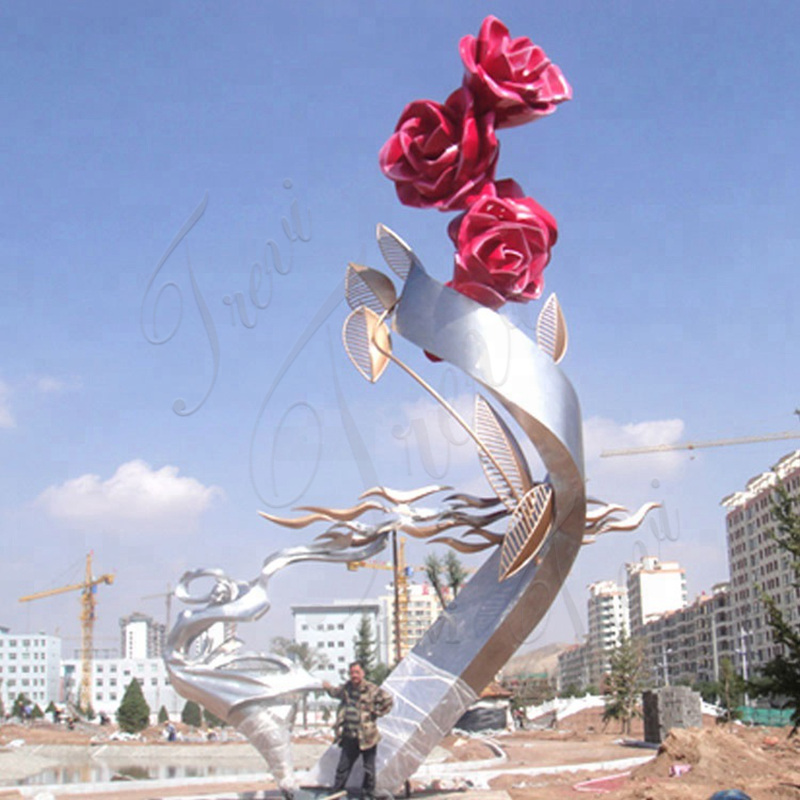In this detailed image, we see a towering, abstract metal sculpture that resembles a twirling dancer adorned with red roses at its peak. The statue is constructed from twisted, silver metal, featuring intricate swirls and ribbon-like elements that lend a dynamic, graceful appearance. In the foreground, a man is striking a feminine pose, wearing black pants, a black and white striped shirt, and a brown army fatigue jacket, with one hand placed on his waist. Behind him, a bustling construction site is evident, with light brown dirt covering the ground, cranes, and a port-a-potty. The backdrop is filled with tall, white commercial or apartment buildings with numerous windows, and above it all, the scene is capped by a blue sky dotted with white clouds.